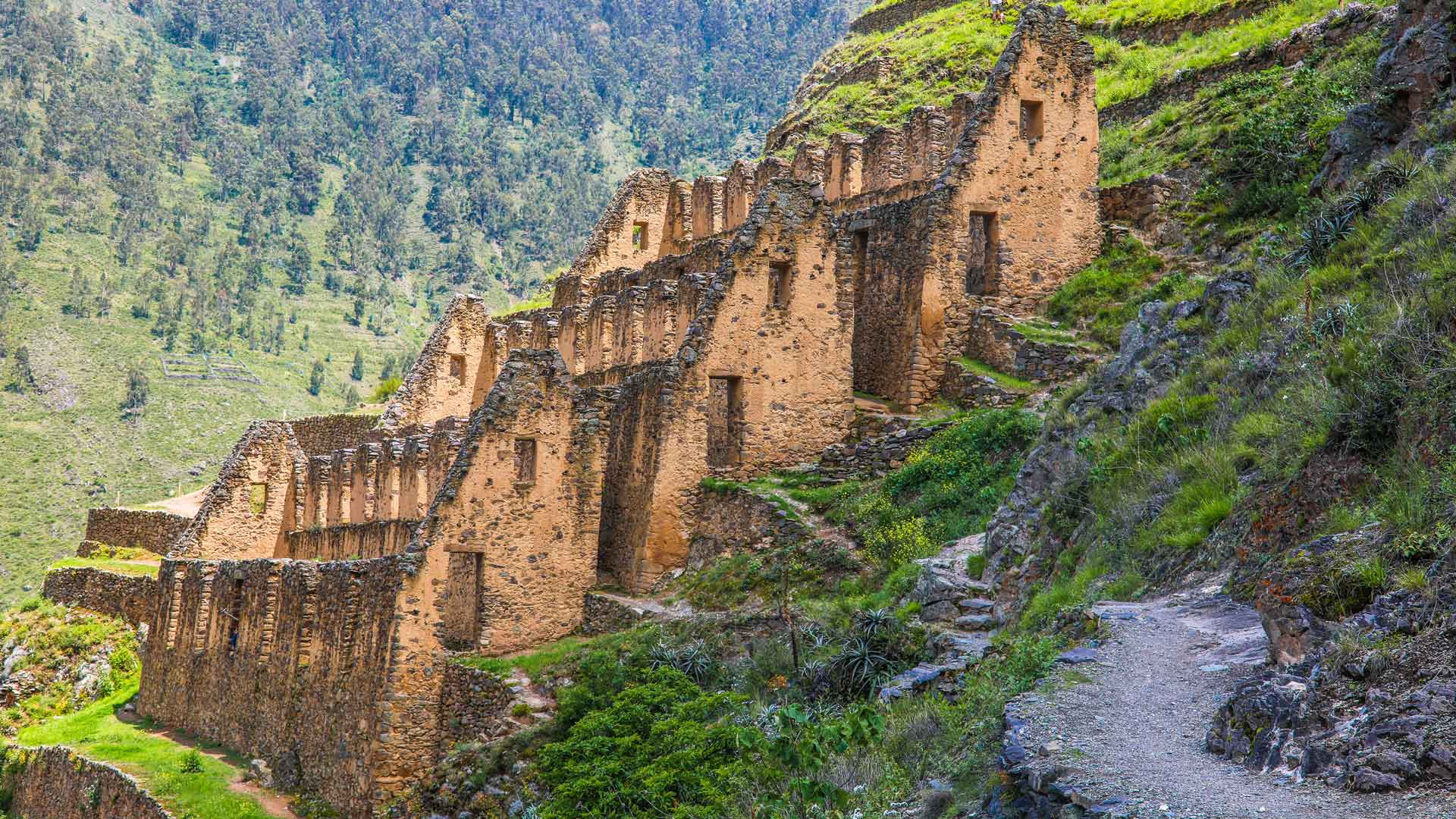The image depicts ancient ruins, possibly of a castle or houses, built into the side of a mountain. The ruins consist of three levels, each resembling distinct sections or houses with exposed infrastructure and stone walls in a sandy brown or light tan color. The structures are devoid of roofs, glass, or doors, and the windows are simply open spaces. The first level has a slope leading to an entryway, suggesting it may have served as a primary entrance. Each subsequent level is set back like steps on the mountainside. Sparse vegetation and faded colors indicate the architecture has been subjected to the elements over many years. The immediate surroundings feature a man-made stone walkway and a path covered with gravel, leading up to the ruins. To the right, you see the continuation of the mountain with green grass growing, while lush greenery, including pine trees, dominates the left side and upper left-hand corner. The overall setting is elevated, under a clear, sunny sky, adding to the serene yet isolated ambiance of this ancient, mountainous landscape.